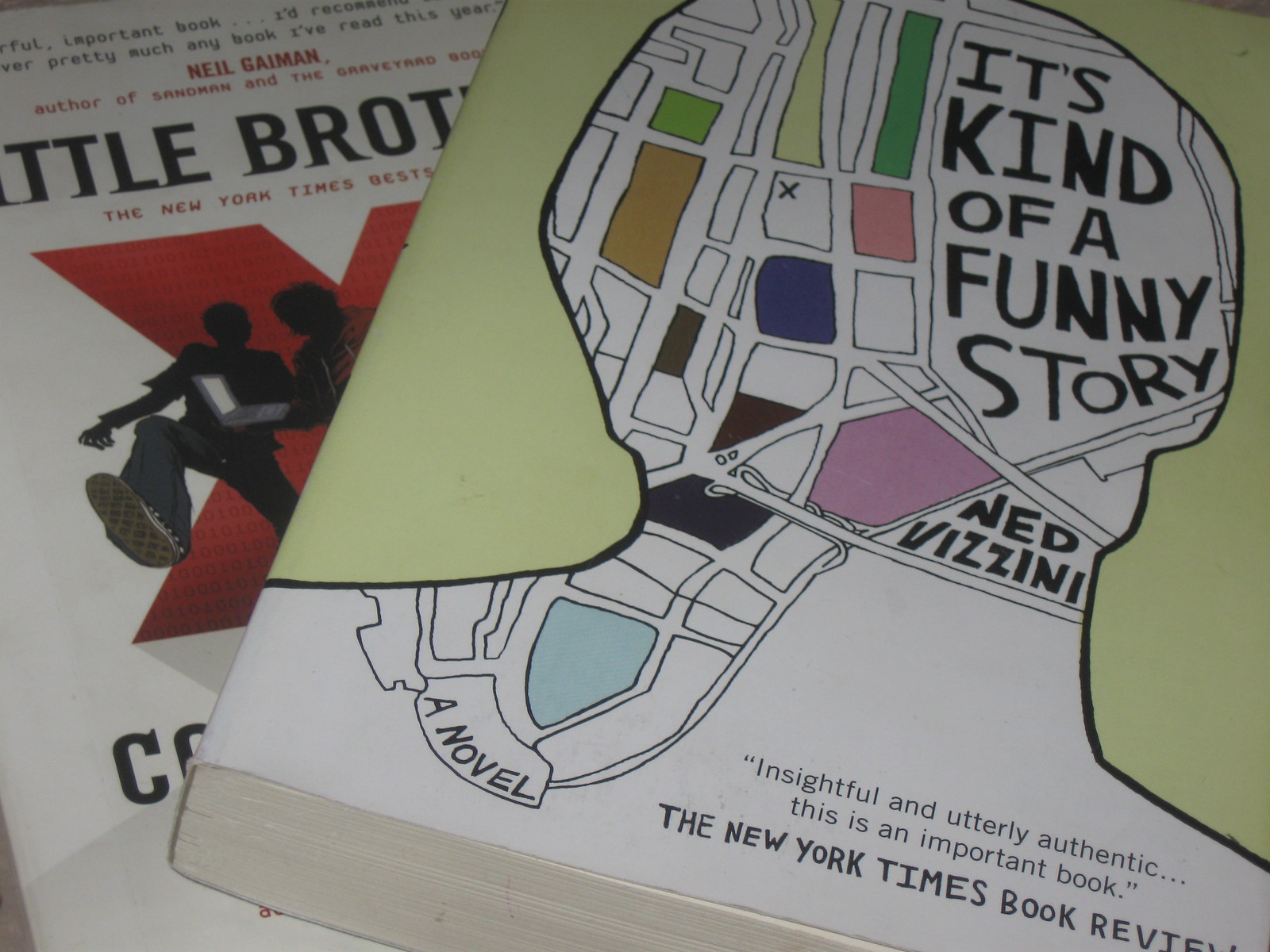This image captures a close-up of two stacks of books positioned one atop the other. The top book, which has a yellow cover, prominently displays the title "It's Kind of a Funny Story" by Ned Vizzini. The cover design features an abstract map, replacing the outline of a person's head, neck, and shoulders with colorful sections reminiscent of a bird's-eye view of a city. These sections are marked by various colors such as brown, green, purple, pink, and blue. Visible within one of these sections is a quote: "Insightful and utterly authentic. This is an important book," noted by a New York Times book review.

Beneath it lies a white book partially obscured, revealing only part of the title, presumably "Little Brother," authored by a writer noted for "Sandman," Neil Gaiman. The cover features a striking red X set against a white backdrop, decorated with coding-like sequences and the silhouettes of two men holding a computer. Additionally, the cover notes it as a New York Times bestseller. Together, these details render a vivid and informative portrayal of the two books in question.